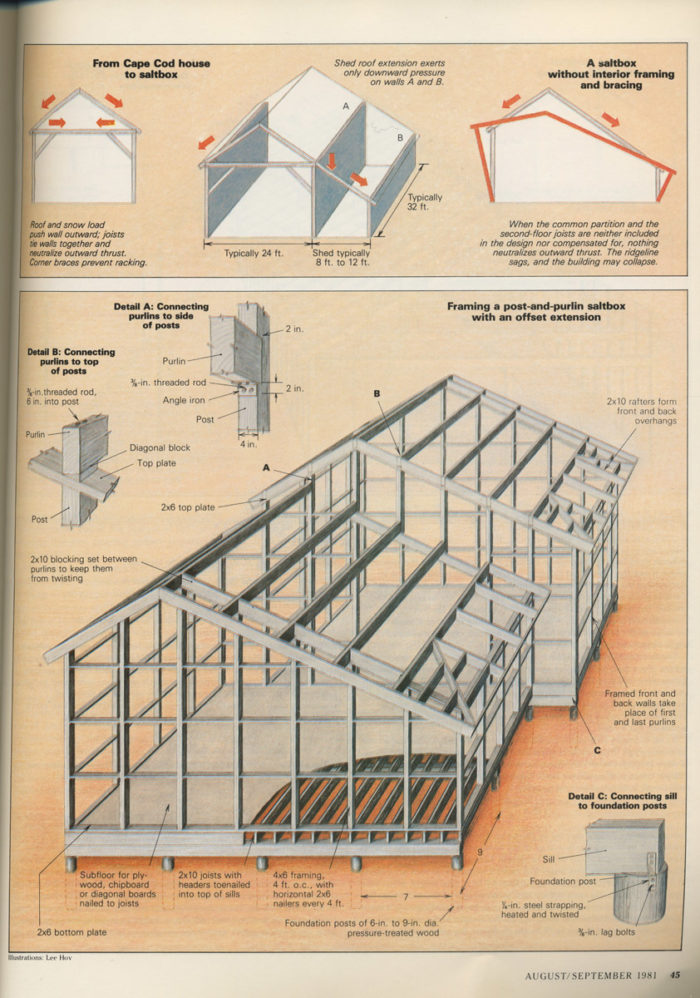This magazine page, dated August-September 1981 and labeled as Page 45, provides a detailed exploration of building construction techniques. The title, "From Cape Cod House to Salt Box," crowns the top of the page, setting the context for the design transformation. An intricate frame construction of a building, devoid of walls or ceiling, occupies the central space. This skeletal structure showcases various building phases and key structural components. 

To the top left and bottom right, close-up illustrations meticulously detail the construction of joints, including the connections of purlins to the tops and sides of posts, as well as the attachment of sill to foundation posts. Accompanying these diagrams are exhaustive verbal descriptions and precise measurements, providing readers with a comprehensive understanding of the construction methods employed.